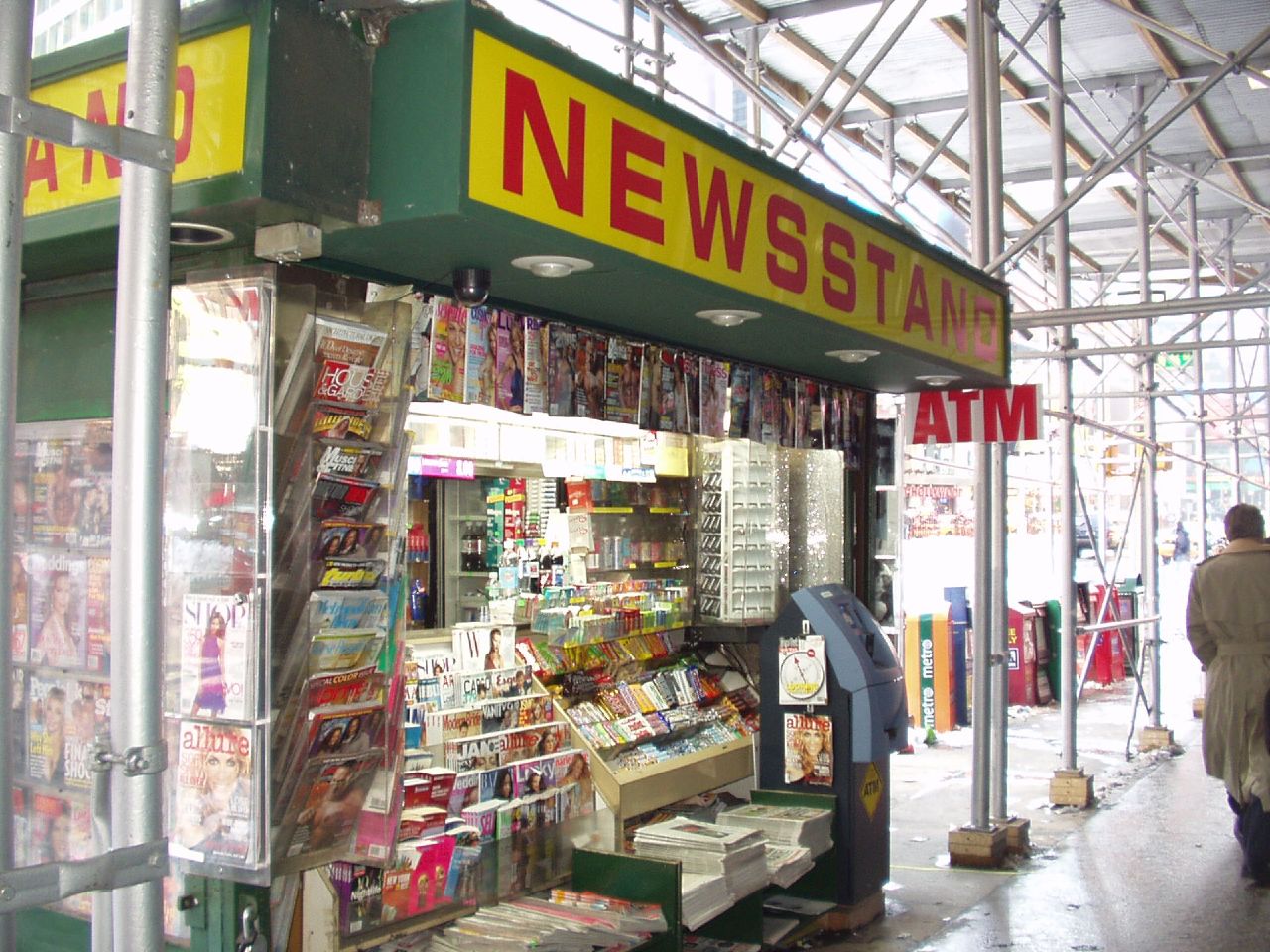In this bustling city street scene, a vibrant green newsstand is prominently featured, standing on a sidewalk and facing towards surrounding buildings. Above the newsstand, a yellow sign with bold red letters spells out "Newsstand," flanked by four lights and a couple of security cameras. The structure is adorned with a multitude of magazines and newspapers, some of which hang across the top and sides, and others displayed on shelves attached to its walls. To the right of the newsstand, blue newspaper vending machines are lined up, and next to them stands an ATM, clearly marked by a red "ATM" sign. Adding to the daily urban hustle, a man in a tan overcoat is captured walking away from the newsstand. Behind the counter, bottles of soda are visible, hinting at the variety of items available for sale. Overhead, an awning supported by metal scaffolding suggests nearby construction or proximity to a transit station or stadium. This quaint, detail-rich snapshot encapsulates a typical newsstand scene, the kind found in major cities worldwide.